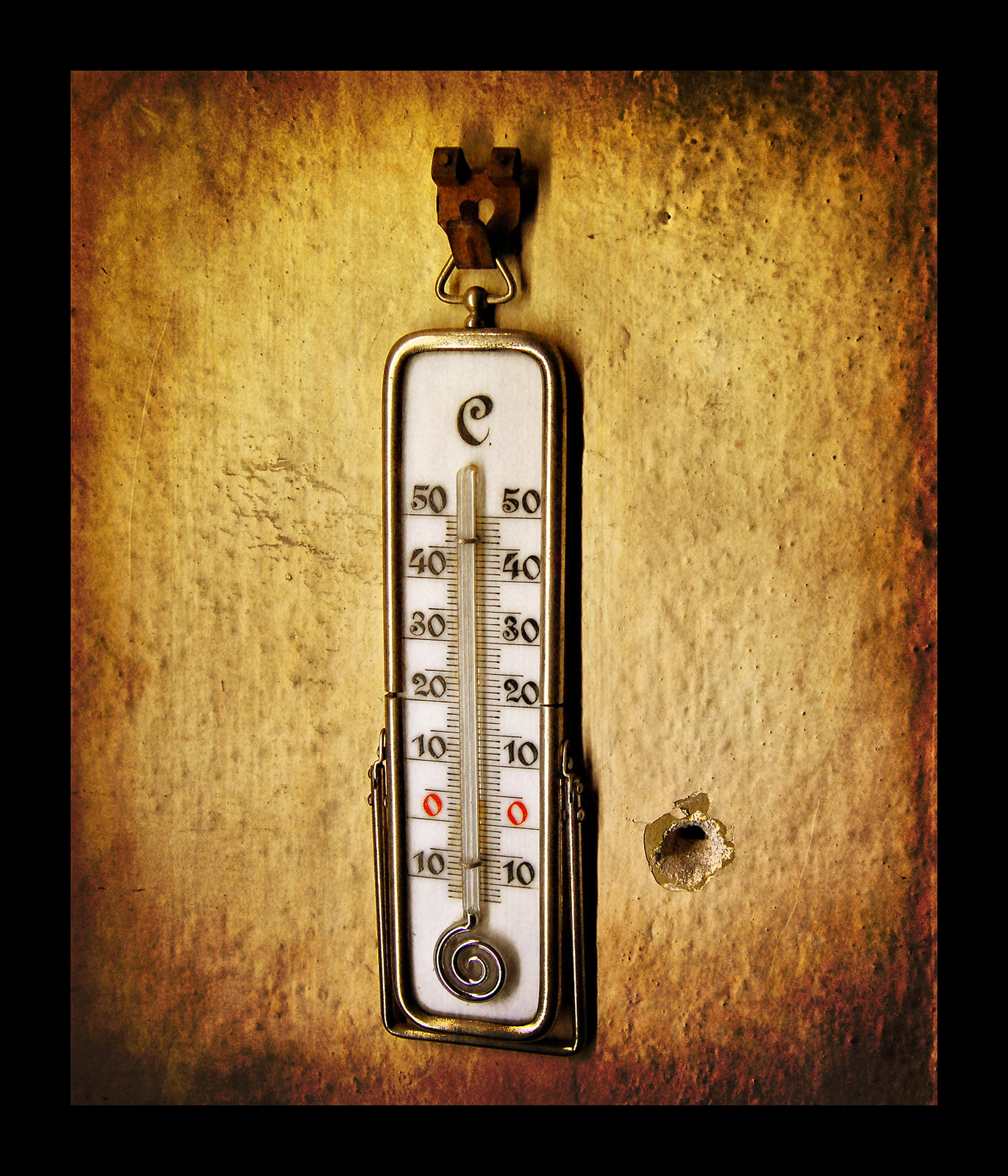The image features an intricate composition bordered by a solid black frame, transitioning into a rustic, dark reddish-orange coloration. This base hue is marred with patches of green and black, eventually fading into a beige-yellow tone on the right side of the image. 

A notable element within this background is a hole, its irregular, jagged edges suggestive of a material akin to drywall. Through this hole, a dark void is visible, enhancing the texture and depth of the surface.

Prominently displayed is an antique thermometer, characterized by its worn-out silver border and an aged appearance. The thermometer is designed with a stand that emerges about a third up from the base, consisting of two brackets leading out to a half-rectangle structure, likely serving as its support.

The thermometer’s white base features a silver, swirl-like pattern at the bottom, which transitions into the cylindrical mercury-filled section used to gauge temperature. Alongside the mercury tube, numeric markings in black font cover the length of the instrument, reading: 10, 10, 00 (with '00' highlighted in red for emphasis), 10, 20, 30, 40, and 50. Crowning the thermometer is an elegant, curly font displaying the letter 'C.'

Each numerical set is neatly separated by thin black dividers, adding clarity and precision to the antique instrument's display.